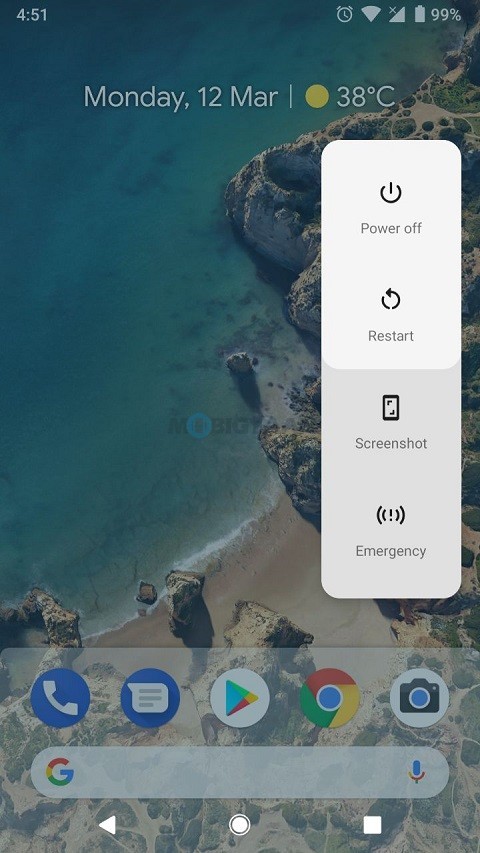The image is a rectangular portrait screenshot from a cell phone, showcasing a beach or waterfront scene from an overhead perspective. The top section of the image features a cell phone interface overlay with the following details:

- **Top Left Corner:** Displays the time in white text, "4:51."
- **Top Right Corner:** Contains five icons, right-justified:
  1. An alarm clock icon.
  2. A solid, diamond-shaped icon resembling a full signal indicator.
  3. A right triangle with its hypotenuse running from the lower left to the upper right, marked with an "X."
  4. A full vertical battery icon with its nub pointing to the top.
  5. A "99%" text indicating a nearly full battery.

**Centered Header:**
- **Top of the Image:** Against a blue water background, the header displays:
  - "Monday, 12 MAR" in white text.
  - A vertical white line.
  - A yellow circle representing the sun.
  - "38°C" in white text with a degree symbol and capital "C."

**Main Image (Background):**
- **Upper 70%:** Blue water with varying shades, resembling a dark aqua color.
- **Border between Water and Land:** An irregular, curvy division with foamy white waves where the water meets the sand and rocks.
- **Lower Right Side:** Rocks transitioning to sand in the lower left corner.

**Overlay to the Right:**
- **Vertical Rectangular Bar (20% down to halfway up, curved corners):**
  - **Top Section (White Background):**
    1. **Power Off:** A power icon with the text "Power off."
    2. **Restart:** A circular arrow icon with the text "Restart."
  - **Bottom Section (Light Gray Background):**
    3. **Screenshot:** A cell phone icon with the text "Screenshot."
    4. **Emergency:** An exclamation point icon with double parentheses around it, labeled "Emergency."

**Bottom Section:**
- **Five Colored Icons (Left to Right):**
  1. Blue circle with a white phone icon.
  2. Blue circle with a white quote box icon.
  3. White circle with a multicolored triangle (Google Play icon).
  4. Multicolored circle (Chrome icon).
  5. White circle with a camera icon with a light blue lens and black body.

- **Search Bar:** Located beneath the icons, white with Google’s colored "G" on the left and a colored microphone icon on the right.

- **Three White Icons at the Very Bottom (Left to Right):**
  1. Left-pointing white triangle.
  2. Filled white circle within a thin white circle.
  3. White square.

This detailed screenshot provides a comprehensive view of the entire interface and a part of the natural landscape below.